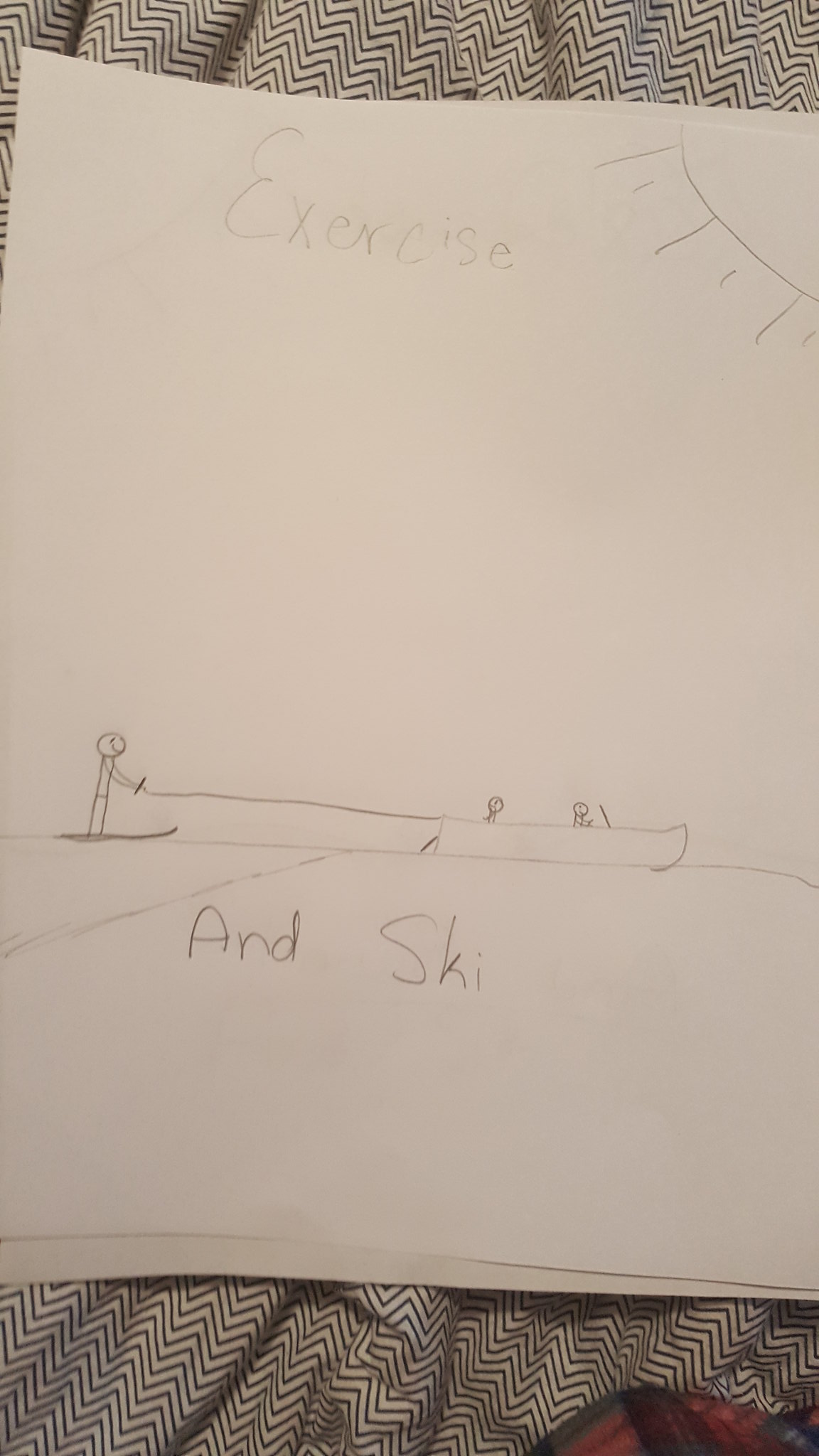This image showcases a piece of drawing paper, which appears to be slightly elongated and blank around the edges. The paper is predominantly white and features what seems to be a child's drawing rendered entirely in pencil. At the top, the word "exercise" is written, with the initial 'E' styled in cursive while the remaining letters are in standard lowercase. In the top corner, there is a simplistic representation of the sun, illustrated with rays extending outward.

The focal point of the drawing depicts a stick figure equipped with skis. This figure is linked by a line, indicative of a tow rope, to a boat containing two additional stick figures. The scene is labeled with the words "& ski.” Below these elements, a horizontal line suggests the presence of water, complete with undulating waves to reinforce the aquatic context of the depiction. The rudimentary nature of the drawing and the whimsical subject matter strongly suggest it was created by a child or a person with limited drawing experience.